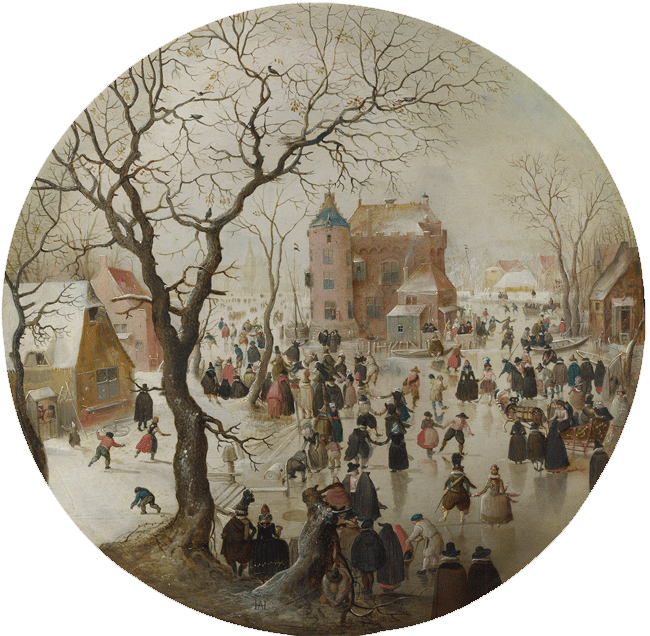This is a circular vintage painting depicting a bustling 19th-century winter scene, reminiscent of an illustration on a Christmas card. The composition features a prominent, leafless tree with a dark brown trunk that stretches to the top edge of the painting. The ground is covered in snow and ice, creating a picturesque setting where children engage in snowball fights, people glide gracefully on ice skates, and sleds, drawn by horses, traverse the wintry landscape. The people, outfitted in a variety of period-specific clothing, including couples holding hands, enhance the painting's charming, bygone-era atmosphere. In the background, Victorian-style buildings and a stone structure with a circular tower and blue conical roof are visible, their red, brown, and dark blue hues muted under a cloudy, moisture-laden winter sky. The scene is imbued with a quaint, old-fashioned ambiance, evoking the feel of a snow-covered village from long ago.